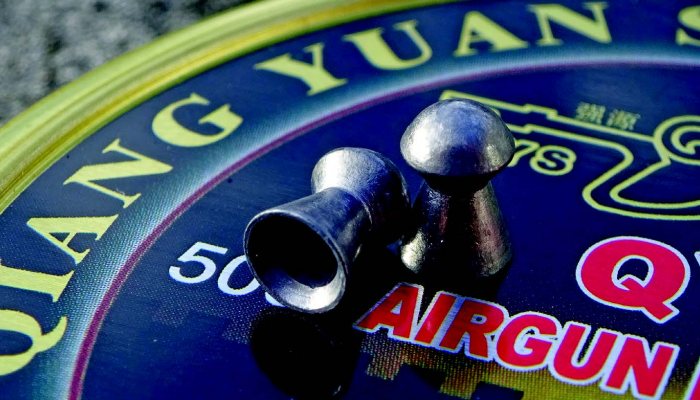The image displays two small, metal airgun pellets with a shiny silver appearance placed on a circular blue lid. The lid, possibly the top of a container, features a yellow rim and has text that reads "Kuang Yuan" and "500 air gun." One pellet stands upright on the right side, while the other lays horizontally on the left. The blue surface includes an illustration of an airgun in yellow, a red "Q" on the lower right, and a partial numerical text "50" slightly visible to the left of the word "air gun." The entire setup rests on a grey surface visible at the upper left portion of the image.